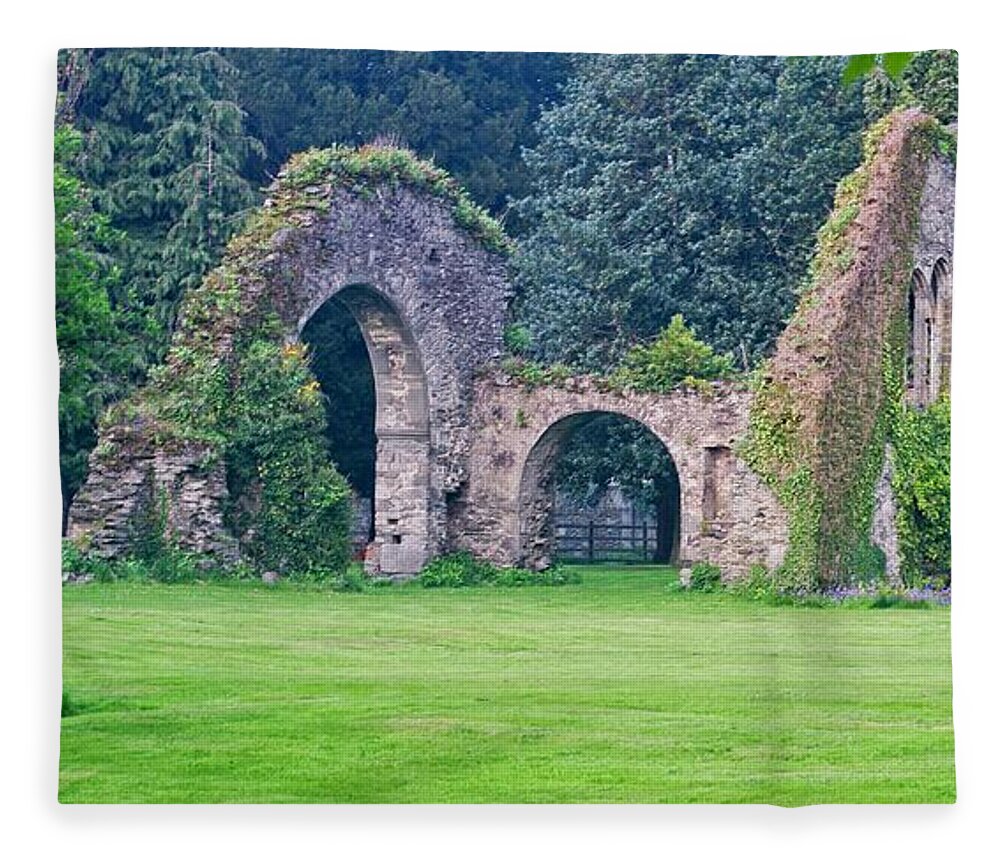The photograph depicts a serene outdoor scene with a well-manicured lawn leading up to the remnants of an old stone structure, possibly part of an ancient castle or building. The ruins consist of multiple stone arches—two prominently positioned ones, along with two additional arches that follow towards the right, suggesting the former grandeur of the edifice. The arches are heavily weathered and overgrown with lush green foliage, vines, and ivy, indicating the passage of time. Algae and other plant life add to the sense of age and abandonment. The foreground features a freshly cut lawn, with a wooden post rail fence running horizontally across the scene. The backdrop reveals a dense forest with a mix of evergreen and deciduous trees, enhancing the natural, untouched atmosphere. The predominant colors in the image are the gray and tan hues of the stonework, contrasted vividly with the vibrant greens of the grass and surrounding vegetation. The entire scene is captured in a photorealistic style, absent of any text.